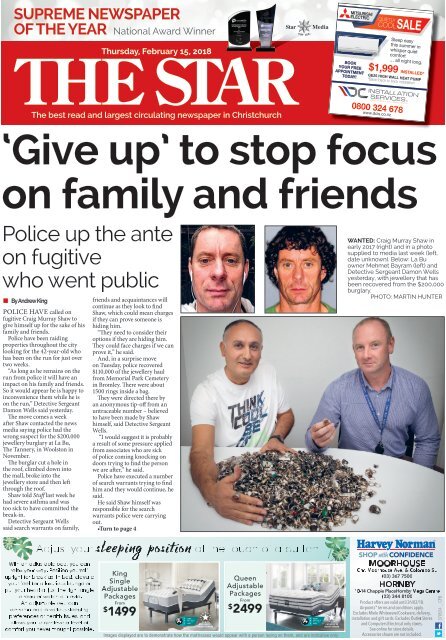The image is a screenshot of an online newspaper website. At the very top, there is a white border. In the upper left corner, a red label reads "Supreme Newspaper of the Year," followed by "National Award Winner." Below that, a red banner prominently displays "The Star" in bold, capital letters. In the upper right of this banner, there is a graphic advertisement for what appears to be a sale on a computer part.

The main article headline reads, "Give Up," in quotation marks, followed by "to Stop Focus on Family and Friends." The article is titled "Police Up the Ante on Fugitive Who Went Public" and is presented in two columns of text.

To the right of the article, there are two images. The first is a more current photograph of a man with very short hair, and the second is an older photograph of the same man with longer hair. Beneath these images, a paragraph is labeled "Wanted." Under this text, there is a large picture of two men sitting at a table, with what appears to be a pile of rocks or other similar objects on the table in front of them.